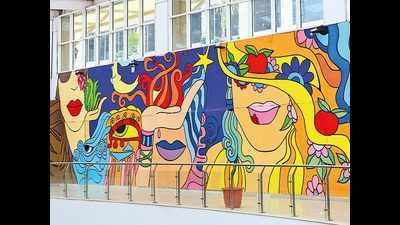The photograph captures a vibrant, colorful mural adorning the lower portion of a building, which contrasts with the upper portion that features a glass wall filled with windows. In front of the building, a tan sidewalk is bordered by a silver railed fence, with a terracotta planter devoid of any plants situated near the bottom of the image. The mural itself, set against a dark blue background, is an abstract and ocean-themed depiction of two women’s faces alongside various other intriguing elements. 

On the left side, there is the partial face of a woman with white skin and brown hair that swirls around her, complemented by large red lips and sunglasses. She holds up her left hand, which reveals red tentacles or flames nestled in her palm. Below her and gazing upwards is a light blue fish with dark eyes and a cranky expression, its tall scales rising above its forehead. An abstract figure with an eye and a mask follows, flanked by a crescent moon. 

In the center of the mural, a figure with red, upright hair and a blue tinge sports purple lipstick and a teardrop beneath the right eye, holding a hand with several bracelets over its eyes. 

On the far right, the mural features the lower portion of the face of a woman with medium-toned skin donning blue and golden yellow hair, pink lipstick, and a yellow sun hat adorned with flowers and apples that obscures the top half of her face. The mural’s vibrant and bold colors evoke a sense of whimsy and surrealism, making it a striking feature against the building’s otherwise modern facade.